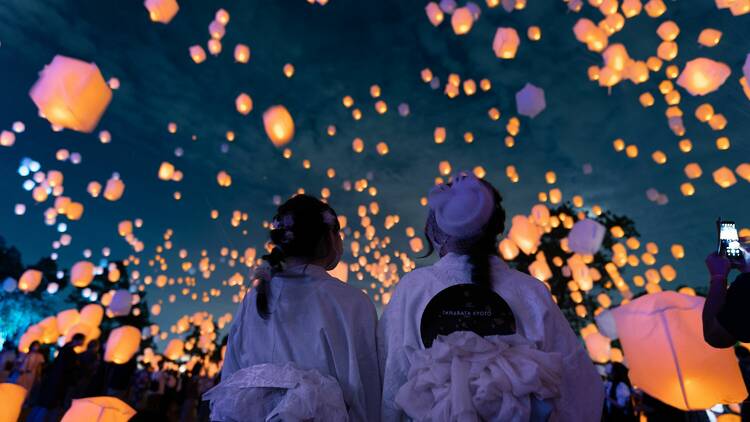The image captures two individuals standing with their backs to the camera, gazing up at an awe-inspiring scene where hundreds of illuminated Japanese paper lanterns float gracefully into the night sky. The lanterns, each powered by a small candle, create a mesmerizing display of glowing orange dots that fade into the distant horizon. The two foreground figures, dressed in white flowing garments with sashes or bows tied at the back, add to the serene and festive atmosphere. One person is adorned with a white cylindrical hat and a black circular emblem on their shirt, though its text is indecipherable. Both individuals have black hair styled in ponytails. To the right, a third person, identifiable only by their long black sleeve and hand, is capturing the moment on a camera phone, underscoring the contemporary nature of the event. The sky, dark yet vividly lit by the numerous lanterns, forms a striking backdrop, while a faint, indistinct crowd can be seen further in the background, enhancing the sense of a shared, communal celebration.